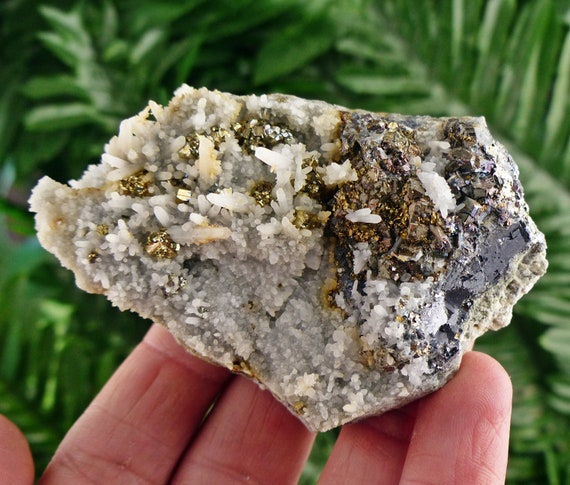In this detailed close-up photograph, a light-skinned individual is admiring a fascinating, uniquely-shaped rock with four fingers—thumb not engaged. The rock itself is a captivating specimen that appears to hail from the ocean, most likely resembling coral or a distinctive cave formation one might find in a gift shop. It's adorned with white crystals sprouting from its surface and showcases a variety of color hues, including black, white, beige, gold, and dark gray. The rock also features several indentations and a salt-like texture, with splatters of brown material, possibly dirt, and a hint of gray clay on one side. The background is dominated by the lush green leaves of a large palm tree, enveloping the entire scene in verdant foliage.